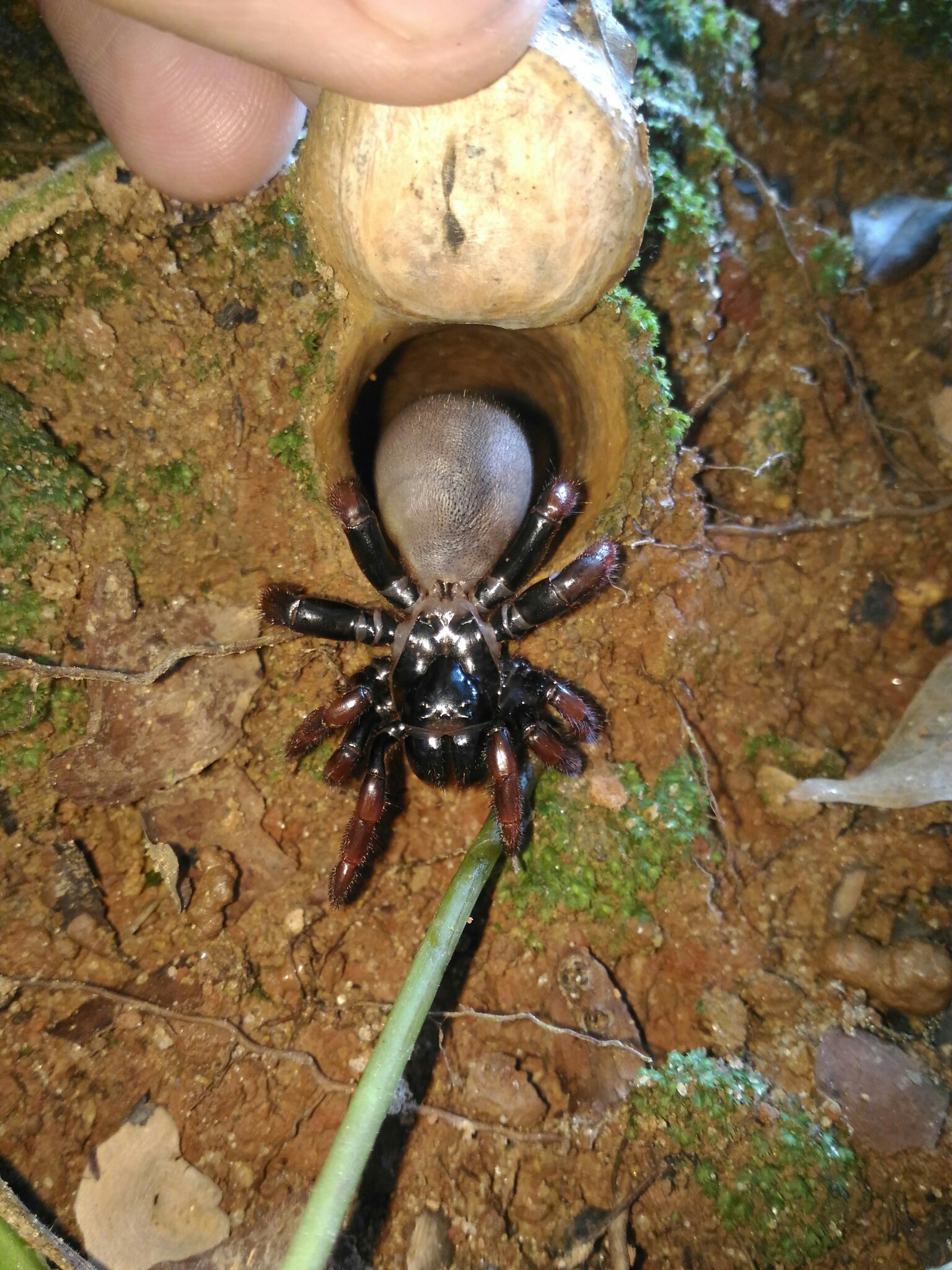This color photograph captures a detailed bird's eye view of a large spider, potentially a wolf spider or a tarantula, situated amidst a natural, earthy habitat. The spider, centered in the image, has a prominent, dark brown abdomen with black towards the middle of its body, and its legs are a furry brown and black. The head of the spider appears lighter in color and features what look like eyes. The ground beneath the spider is muddy, interspersed with dead leaves, small rocks, patches of green moss, and a little grass, enhancing the natural setting. 

In the upper part of the image, an index finger and a thumb intrude slightly into the frame, holding up an unidentified silver object, perhaps some kind of nest or structure related to the spider. Meanwhile, at the bottom of the frame, a green stick appears to be coaxing or interacting with the spider. The intricate details of the spider are clear, highlighting its entire body and eight legs, creating a striking contrast against the earthy background.